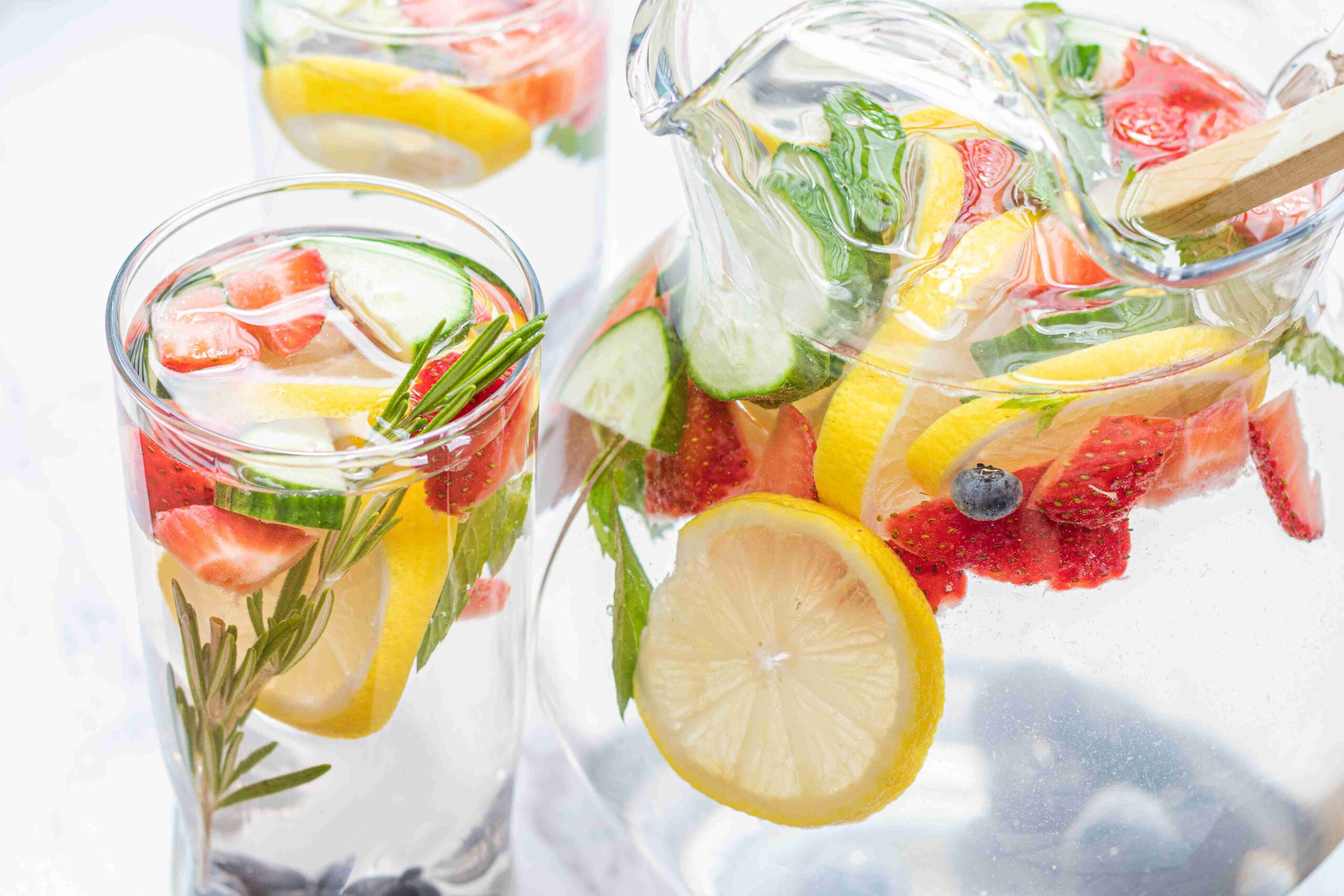This detailed photograph features a clear glass pitcher and two glasses filled with fruit-infused water set against a white background, which highlights the vibrant colors of the ingredients. The pitcher dominates the right two-thirds of the image and contains a mix of clear liquid—likely water, but possibly alcohol—infused with two lemon slices, five strawberries, one halved piece of cucumber, a couple of blueberries, and long sprigs of herbs, likely mint and rosemary. A wooden spoon, used for stirring, is visible entering the pitcher from the top right, with its handle jutting out of the frame. To the left of the pitcher, a glass in the foreground shares the same colorful mix of fruits: lemon slices, strawberries, cucumber halves, rosemary, and mint leaves. This glass notably lacks blueberries. Farther back, a second glass shows fewer fruits, but unmistakably contains lemon slices, strawberries, and mint leaves, maintaining the consistency of the refreshing mixture. This inviting scene captures a visually appealing and delicious setup of fruit-infused water.